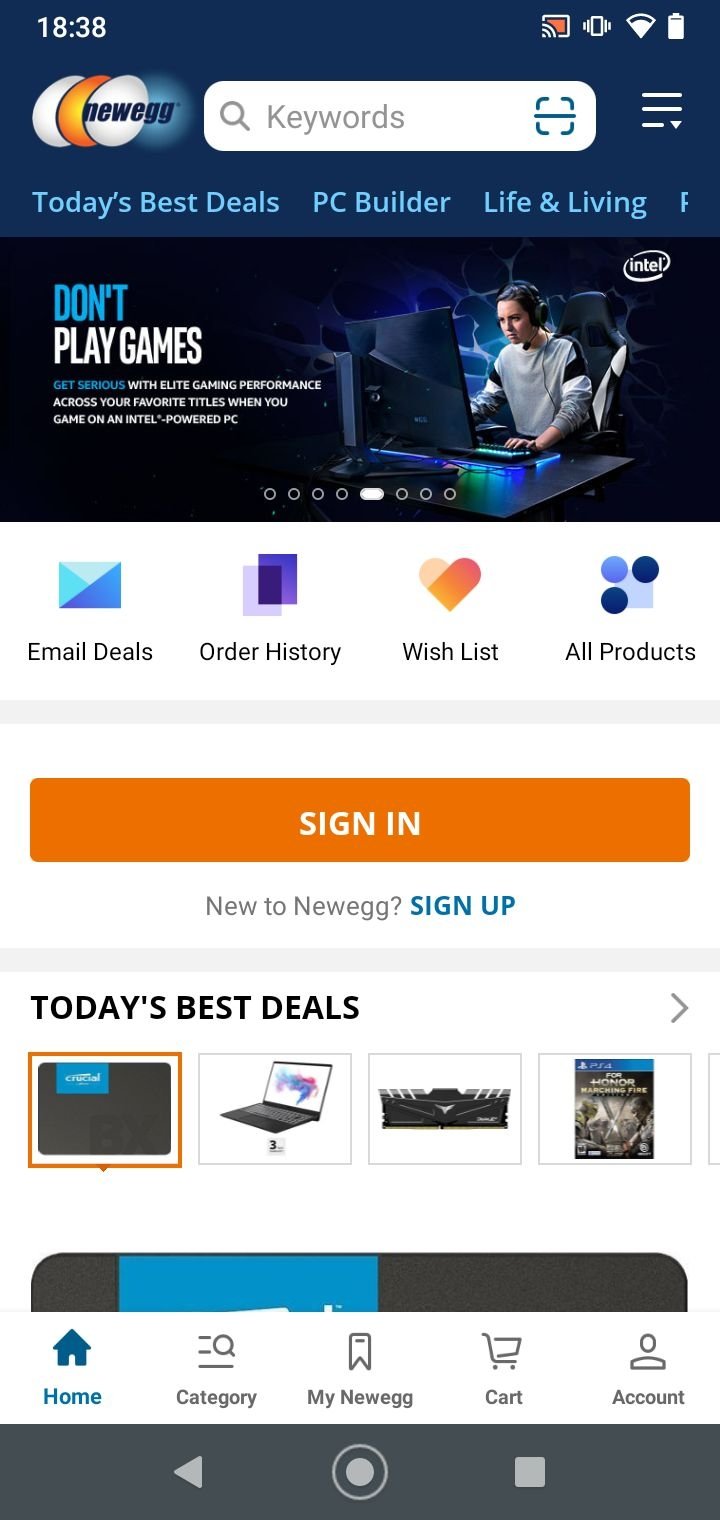This screenshot captures the mobile view of the Newegg website. At the very top of the image, the phone status bar displays the current time, Wi-Fi signal strength, and battery level. Below this, a dark blue header features the Newegg logo, comprising the word "Newegg" encased within stylized egg shapes of varying colors. Directly to the right of the logo is a searchable keyword bar, followed by a navigation bar offering quick access to various site sections.

Beneath this navigational header are three prominent hyperlinks titled "Today's Best Deals," "PC Builder," and "Life and Living." Below these links, the central part of the screen features an image of a person engrossed in a desktop gaming setup, complete with a light-up keyboard and dual monitors. Accompanying the image is a bold text that reads "Don't Play Games," with smaller text underneath that is illegible due to its size.

Following this dark blue section, the site layout transitions to a white background. Here, four navigational links are provided for "Email Deals," "Order History," "Wish List," and "All Products," each paired with corresponding icons. A prominent orange hyperlink bar labeled "Sign In" stands out in white text, and directly beneath it, a blue clickable link reads "Sign Up" next to the phrase "Nude at Newegg."

Further down, the section titled "Today's Deals" showcases four featured products, though the specifics are unclear due to the distance from the viewer's perspective. These appear to include a laptop, a keyboard, and a video game. The screen continues to a second navigation bar with options for "Home," "Category," "Newegg," "Cart," and "Account." Here, the "Home" icon is highlighted in blue, while the other options are shown in faint gray against a white background.

The bottom of the screenshot is occupied by a dark gray strip displaying white icons for navigating the phone's interface.